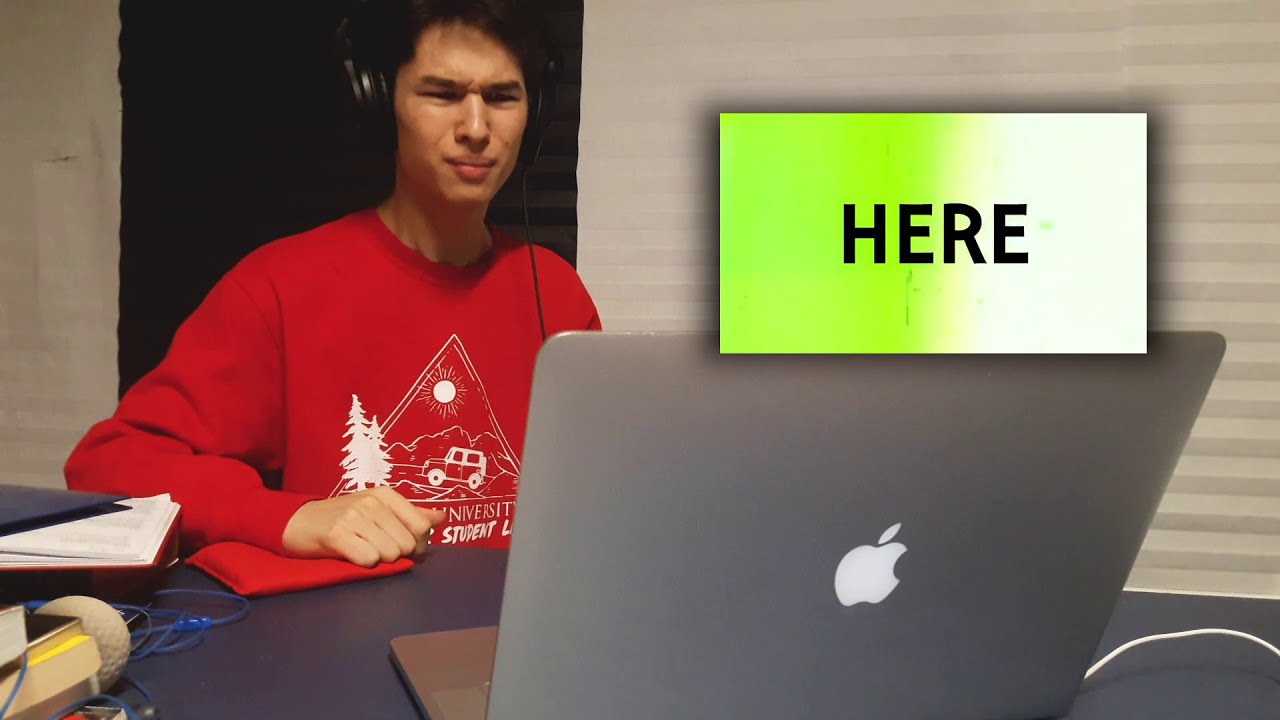The photograph features a man of likely East Asian descent, positioned towards the middle left-hand side of the image, sitting at a gray table. He has short, dark hair and is wearing black headphones, with the right headphone not visible. The man is dressed in a red long-sleeve sweatshirt adorned with a white triangular design, accompanied by images of trees, a sun, and possibly a car. The sweatshirt also has the words "university student" printed in white. His right hand rests on a red object that resembles a pencil case or mouse pad, while various papers or books are scattered to his left. In front of him on the table is an open Apple laptop, bearing the distinctive silver casing and Apple logo. He appears to be squinting at the laptop screen. Above the laptop, there is a white rectangle with the word "HERE" in black capital letters; the rectangle has a green background on the left side and a white background on the right. The background behind the man features a gray wall with darker horizontal stripes, and a black door that is slightly blurred. Additionally, a white cord connected to the laptop extends off to the right.